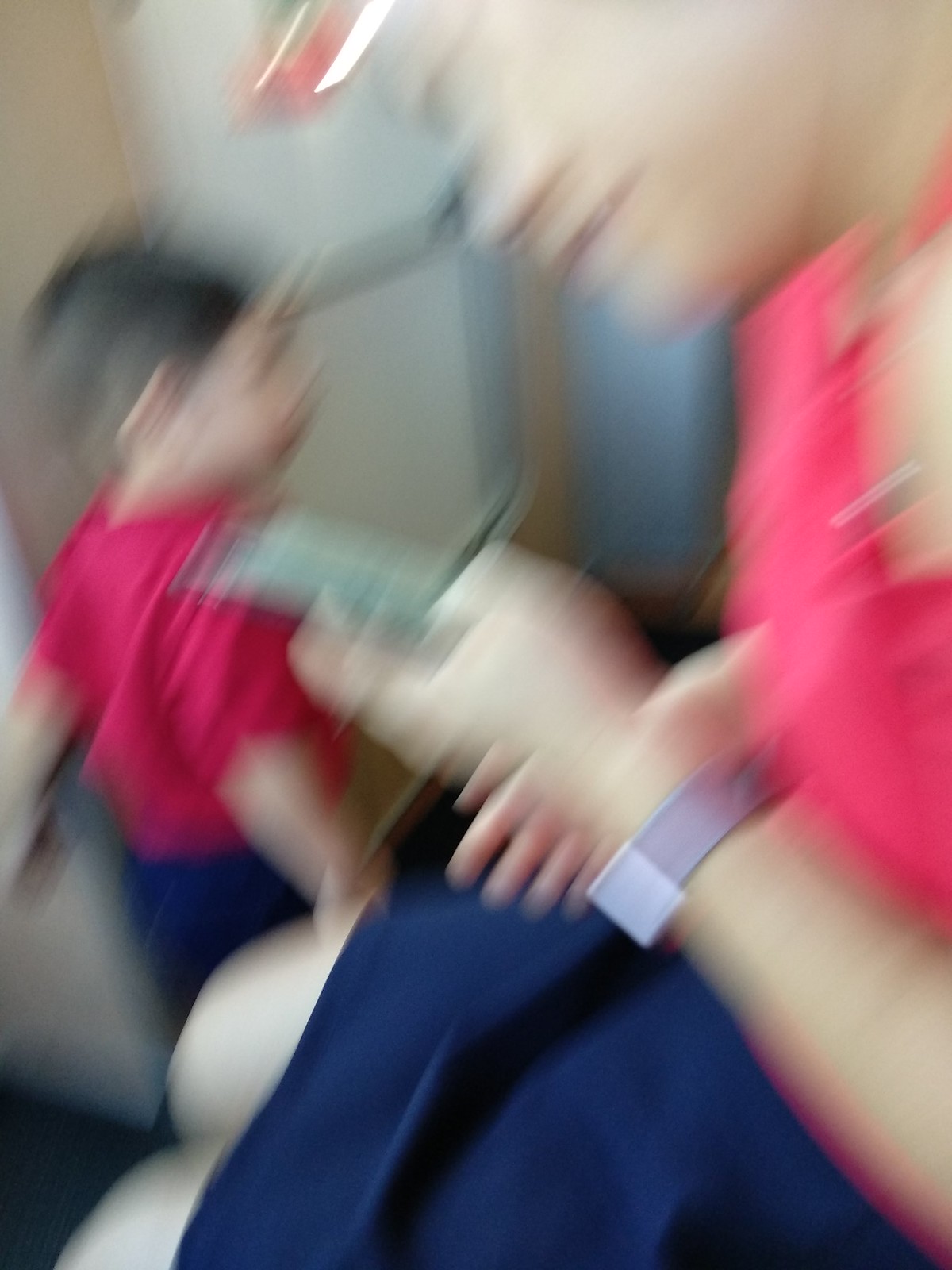In this blurry, vertically-oriented photograph, the focal point is a lady on the bottom right side of the image, captured in profile as she looks at her smartphone. She is wearing a sleeveless red shirt and a blue skirt, complemented by a gray wristband that appears to be a smartwatch on her left wrist. The lady is seated, with part of her knees visible in the foreground. Sharing the frame is a young boy, approximately two or three years old, with short brown hair and light skin. He is dressed in a red T-shirt with short sleeves and blue pants, and seems to be walking away from her. Both figures are set against a background that could possibly be a room with beige walls, featuring a white refrigerator and a blue trash can, although the details are very hard to discern due to the overall blurriness of the image. The photo's indistinct nature gives it a sense of motion, leading some to speculate that it might have been taken inside a moving vehicle, such as a bus or a train.